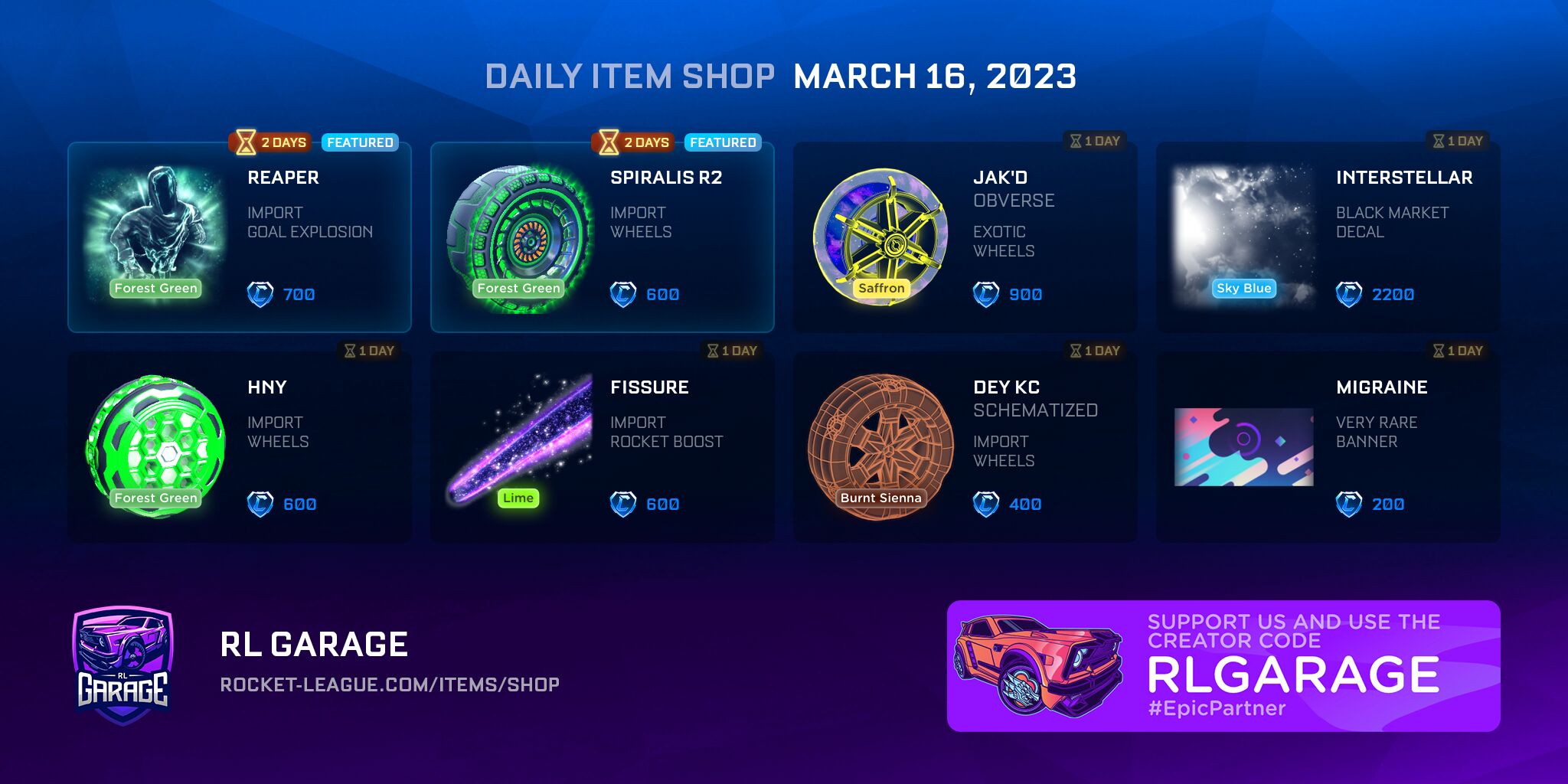In the image, we see a vibrant, dynamic scene that appears to be a screenshot from a mobile game interface. The aspect ratio of the image is approximately 2.5 times wider than it is tall. The background presents a gradient of colors, starting with a lighter blue at the top, transitioning through darker blues in the middle, and finally blending into a purplish hue towards the bottom.

In the foreground, eight rectangular icons are arranged in a grid, four icons wide and two icons deep. Each icon represents an item available for purchase within the game, accompanied by a small blue gem icon and a price tag denoting the cost in virtual currency. Prices vary, ranging from $600 to $900, with the value seemingly increasing from left to right.

The first icon showcases a character named "Reaper," depicted as a figure reminiscent of Iceman but adorned in teal. The second icon is labeled "Viralist R2," featuring a green wheel-like design. The third, titled "Jax'd" (J-A-K apostrophe D), displays a blue circle with yellow spokes at its center. The fourth icon, named "Interstellar," depicts a storm cloud, hinting at a celestial or weather-related theme.

Overall, the image is a detailed snapshot of the game's in-app store, where various characters and items can be acquired, each with distinct visual representations and prices.